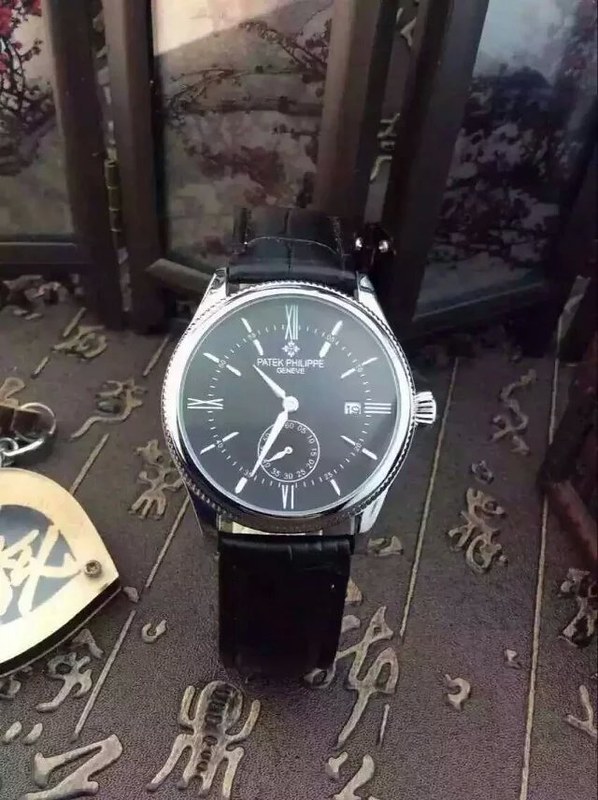The photograph features a luxurious wristwatch, elegantly displayed on a richly ornate dresser surface. The surface is adorned with intricate gold writing and lines that run the length, adding a touch of opulence. The watch boasts a sophisticated black leather strap, complementing its bright silver, almost white, watch face. The face itself is black, marked with refined Roman numerals that indicate the time, which is approximately 10:35. The watch includes a smaller inset clock face for tracking seconds, and a silver winding dial on the side. In the background, delicate screen paintings with a floral design, possibly of Asian influence, enhance the image with additional depth and cultural texture.